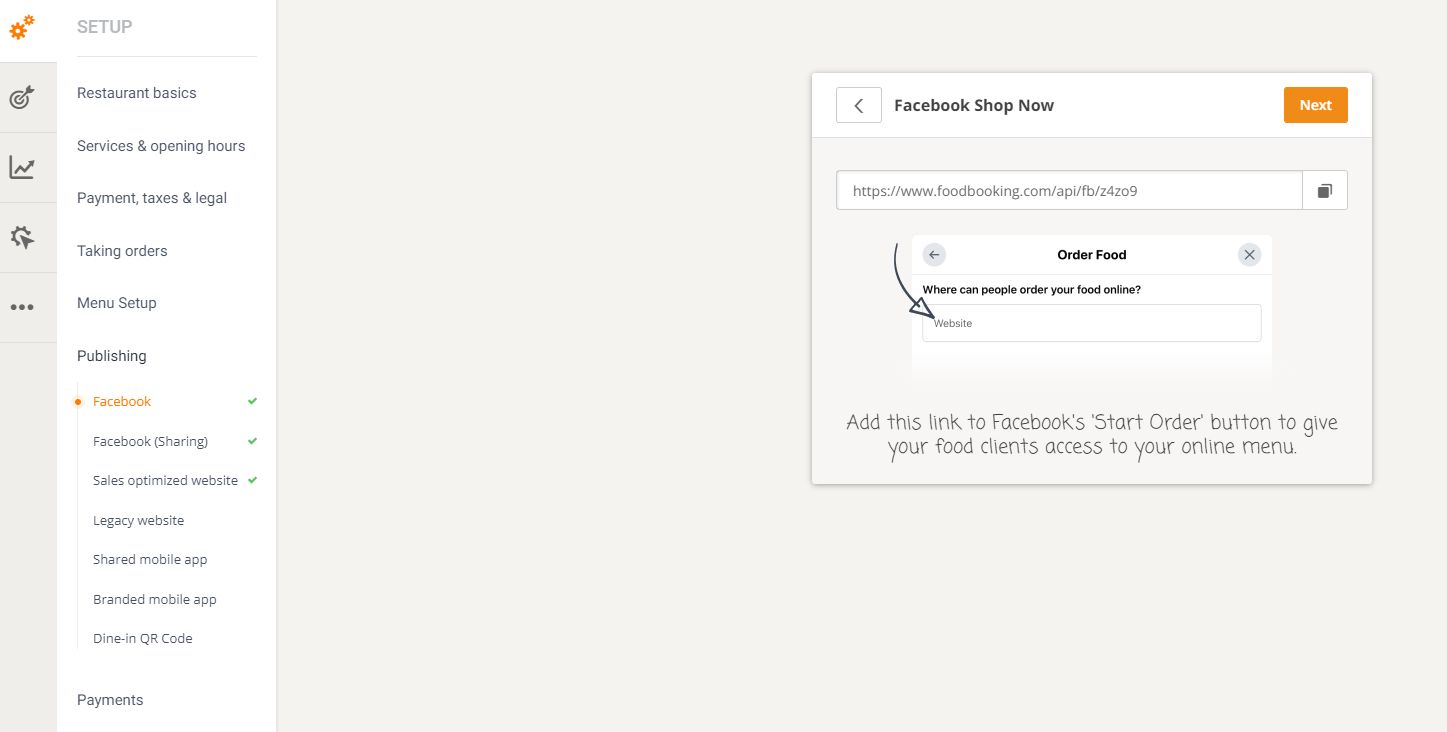In the image, there is a detailed user interface related to setting up an online food ordering system for a restaurant. On the right side, there's a square, approximately five inches in length, with a small arrow pointing to the left. Next to it, the text "Facebook shop now" is visible. Further right, inside an orange rectangle, there's the word "Next."

Adjacent to that, there's an open search bar with a downward-pointing arrow labeled "Order food." The search bar is highlighted for users to enter their queries, accompanied by a prompt that says, "Where can people order food online?" Below the search bar, there's a message instructing users to "Add this link to Facebook's start order button to give your food clients access to your online menu."

On the left side of the image, an orange circle is displayed next to the word "Setup." Below "Setup," a list of menu options is presented, including "Restaurant basics," "Services and opening hours," "Payment, taxes, and legal," "Taking orders," "Menu setup," "Publishing," and more. Each menu option is accompanied by an orange circle indicator. Additional features listed include "Facebook sharing," "Sales optimized," a "Shared mobile app," a "Branded mobile app," and "Dine-in QR codes."

Finally, about two inches down from these options, there's the word "Payments," indicating another section of the setup process.